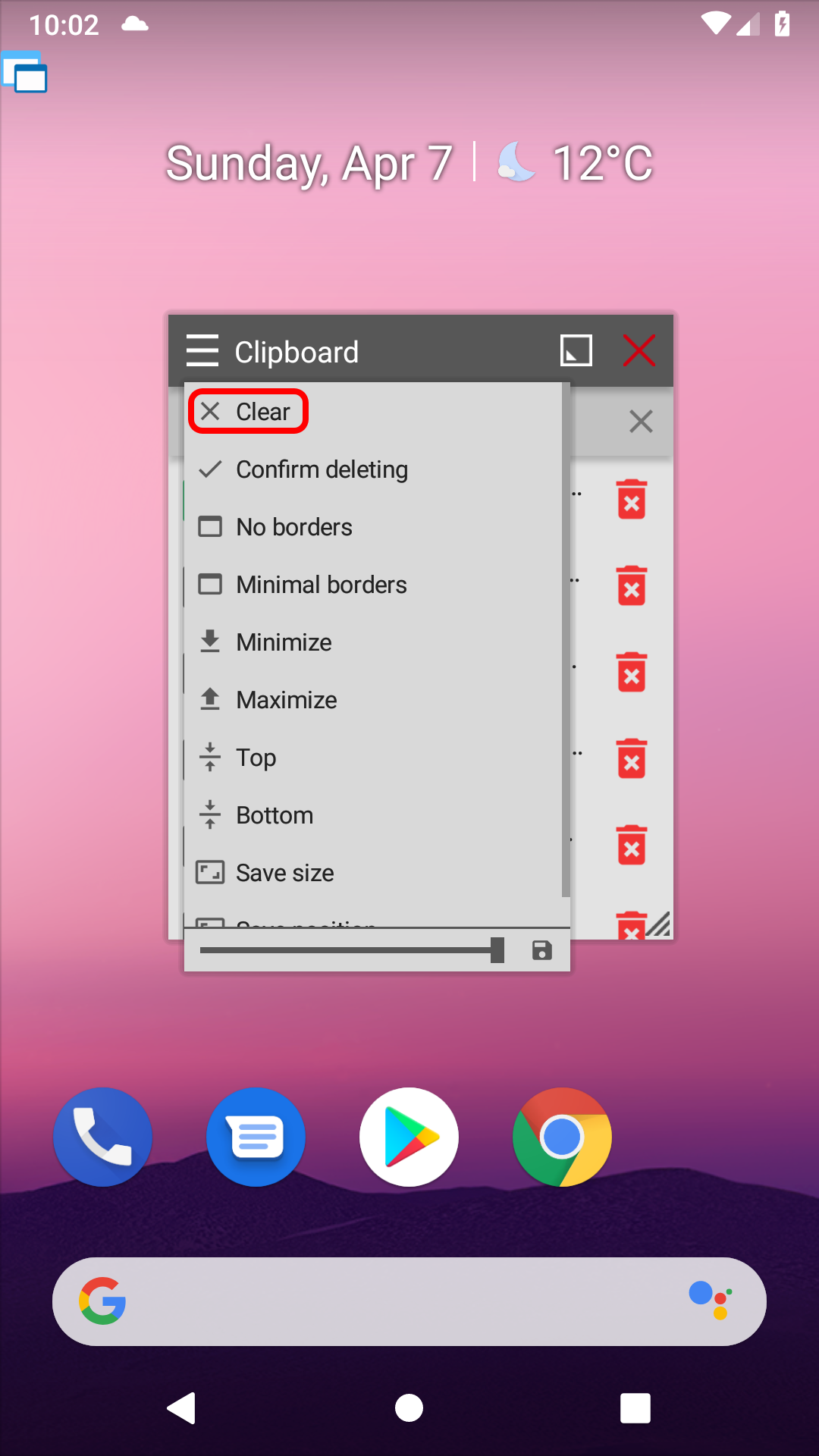The image is a detailed view of a cell phone screen. At the very top left corner, the time is displayed as "10:02" with a cloudy weather icon beside it. The status indicators, including cell signal bars, Wi-Fi connectivity, and a charging battery icon, are all depicted in white.

Centered on the screen, the date "Sunday, April 7th," along with "nighttime" and a temperature of "12 degrees Celsius," is displayed prominently. Below this, a pop-up menu titled "Clipboard" appears with a menu pulled out, featuring options listed in a pull-down format. Within this menu, the option "X, clear" is highlighted by a red circle.

Continuing down, the pop-up menu lists additional options: "Confirming," "Deleting," "No Border," "Minimal Border," "Minimize," "Maximize," "Top," "Bottom," and "Save Size." Behind this pop-up, another instance of the "Clipboard" menu is faintly visible but largely obscured. On the right side of the screen, there are multiple red garbage can icons, and a visible red "X" icon is used to close the menu.

Further down the screen, icons for essential applications are displayed: Phone, Text, Google Play Store, and Google. A Google search bar is situated below these app icons. At the very bottom, navigation buttons for the phone—left arrow, circle, and square—are aligned.

The background wallpaper of the cell phone starts at the bottom with deep purple, almost black hills. From these hills, the gradient transitions smoothly from light purple to dark pink as it moves upwards, culminating in a light pink at the top, where the cell phone information is displayed.